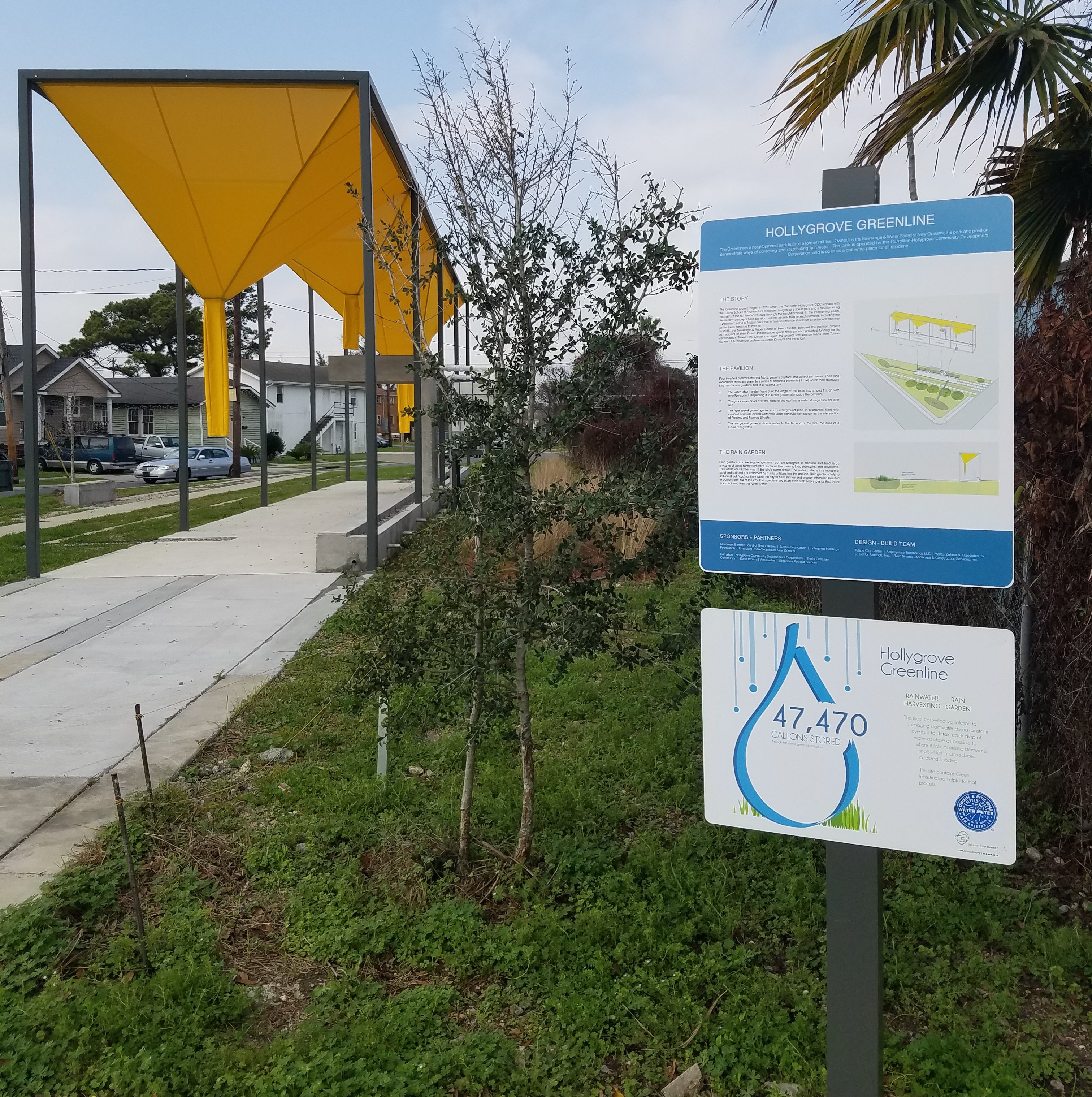This image captures a neighborhood featuring the Holly Grove Greenline, a dedicated area focused on water conservation and environmental preservation. In the foreground, multiple signs explain the Greenline initiative. The primary sign reads "Holly Grove Greenline" and includes images and text detailing its water storage capacity of 470 gallons, with a smaller accompanying sign providing additional information. Both signs are mounted on dark wood stakes. The landscape showcases a lush, green environment with ample grass and bushes, and a slender tree takes center stage.

To the left of the image, there’s an interesting yellow structure resembling a canopy or tent, designed with vertical metal bars that support the fabric. This canopy, which may serve a practical role in water collection or rain coverage, is positioned above a straight sidewalk running through the grassy area. In the background, large homes with parked cars in driveways and garages are visible, under a clear blue sky with a small patch of clouds. This scene illustrates a harmonious blend of residential life and eco-friendly initiatives within the Holly Grove Greenline area.